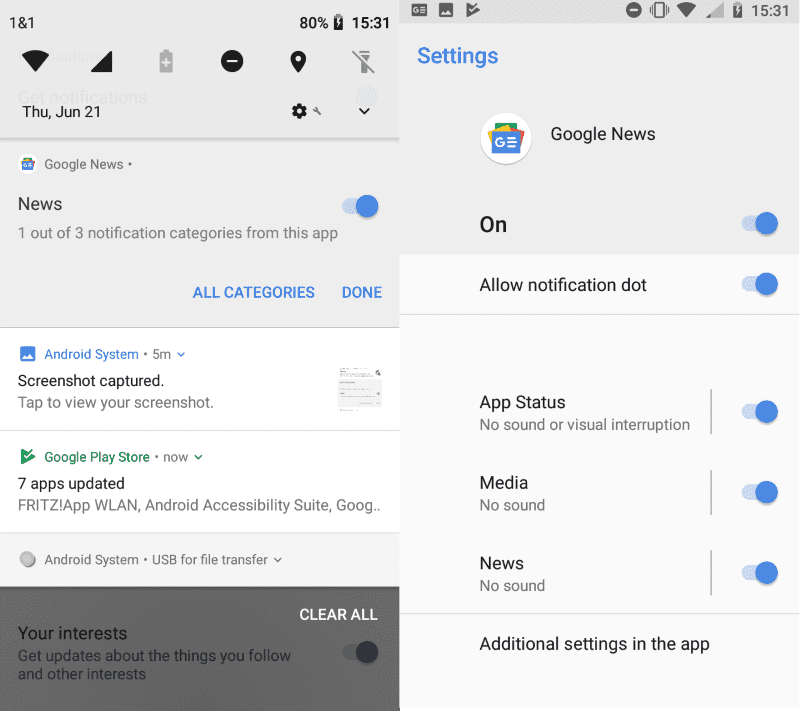The provided image consists of two smartphone screenshots placed side-by-side, both taken at the same time—15:31—as indicated in the upper right-hand corners, accompanied by battery symbols. 

In the left screenshot, the battery level is displayed at 80%, while the right screenshot displays additional icons such as Wi-Fi and cell signal indicators, but not the battery percentage. The left screenshot showcases a typical Android notification panel with the date "Thursday, June 21st" and several notifications. Among these, Google News indicates one out of three notifications, another from the Android system states that a screenshot was captured five minutes prior, and a Google Play Store notification mentions that seven apps have been updated. 

Meanwhile, the right screenshot delves into the settings for Google News notifications, where options to toggle notifications for 'app status,' 'media,' and 'news' are all currently enabled. It appears the user might be adjusting these settings, potentially aiming to disable notifications from Google News. 

These two screenshots collectively illustrate routine interactions with an Android phone's notification management and settings adjustment features.